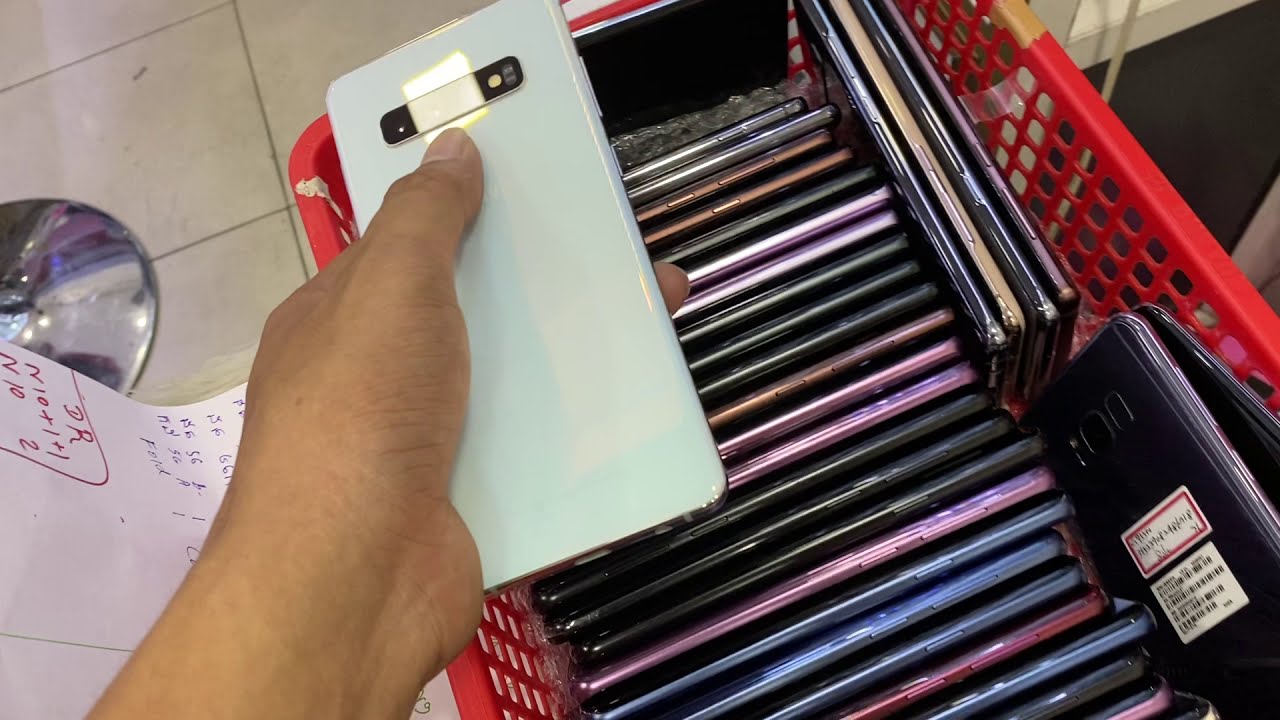In the image, a close-up shot captures a tanned left hand holding a white smartphone with a small black magnet attached to its back, positioned over a red plastic handbasket. The basket, reminiscent of those used in grocery stores, is filled with an assortment of smartphones in various colors, including purple, blue, burgundy, black, gold, and white. Among the smartphones, there is a distinct black flip phone at the bottom right, adorned with two white stickers below its camera area. To the left of the hand, a white sheet of paper with numbers written on it is visible, featuring a top box in red marked with "1, R, N10, plus 1, plus 1, N10, and 2" on the next line. Additional numbers written in blue can be seen, though partially obscured and bent into a C shape. The upper left corner of the image reveals a glimpse of the tile flooring and a silver round piece, potentially part of the queue management poles of the business setting.